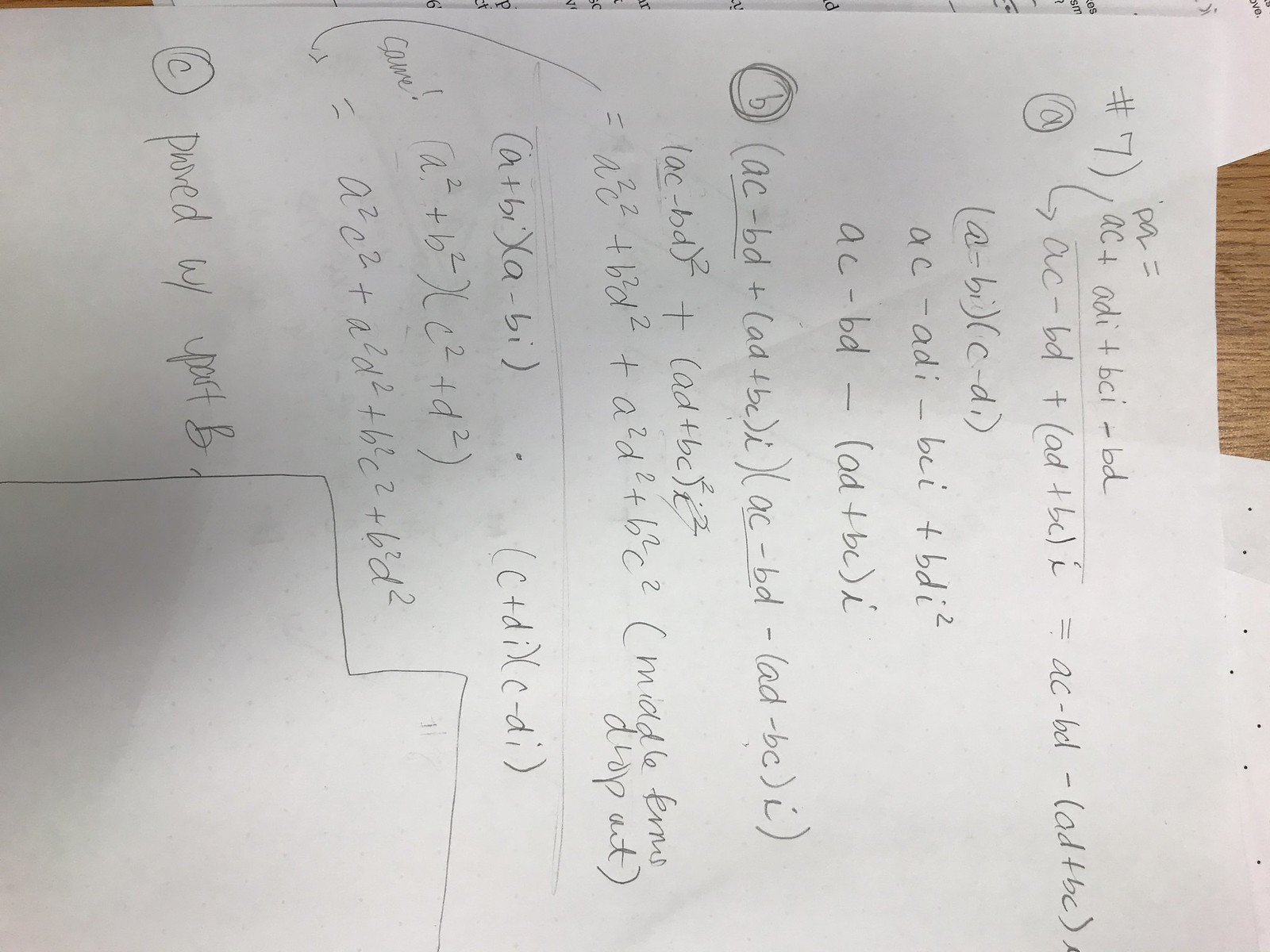This image depicts a piece of paper oriented horizontally, showcasing what appears to be algebra homework. The top of the page is aligned to the right, and the bottom is on the left, with the writing flowing from top to bottom along the right edge of the paper. The text on the sheet is printed sideways, with the tops of the letters pointing to the right and the bottoms pointing to the left.

The main sheet overlaps a smaller fragment of paper that comes in from the top right, extends downward about an inch, and then angles upward and off the right side. A wooden surface, approximately two inches wide, is visible at the bottom of the image. Below this, there is another piece of white paper under the main sheet, slightly angled downward towards the left and then downward towards the right.

On the algebra homework, there are three numbered problems. The first, labeled as 7a, includes the equation \(7a(B - DC) = X^2\). Below this, problem 7b can be seen, and a third problem is partially visible beneath 7b, though its contents are obscured. The bottom left, which in the rotated orientation is the bottom of the page, contains the instruction "prove W/part B". 

Additionally, a line enters from the left side of the page, extending roughly three inches before descending about two inches, continuing horizontally to the right for about an inch, and then dropping off the bottom edge of the page.